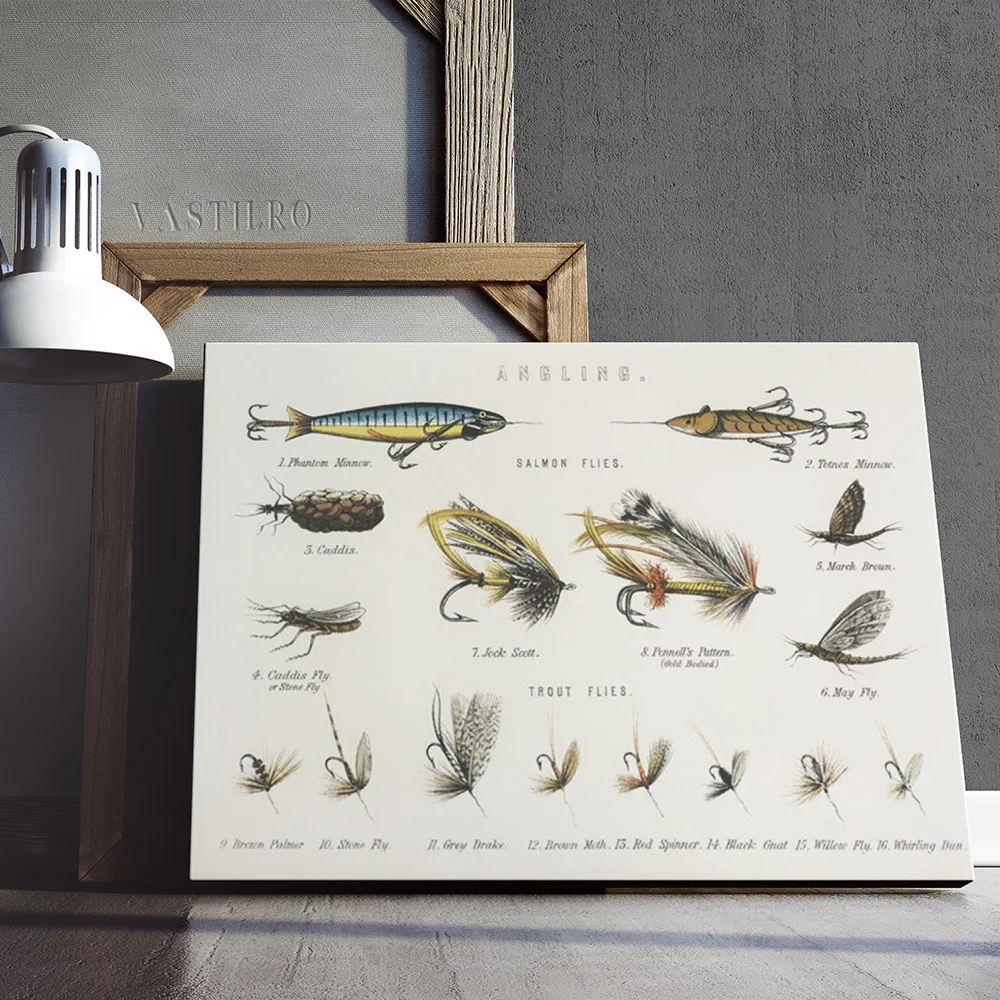In the photograph, an indoor scene is depicted featuring a gray-painted cement wall with a white baseboard along the bottom edge. The wall is divided by a lighter gray vertical stripe down the center, with a slight indentation on the left side spelling out "V-A-S-T-I-L-R-O." Resting on the brown wooden floor, in front of the wall, is a small, white desk lamp positioned on the top left side of the image. Moving to the right, there is a large, beige wooden-framed picture frame, slightly ajar, revealing a glimpse of the gray wall behind it. In front of this, there is a smaller, light brown wooden-framed picture leaning against the larger frame.

Dominating the foreground is a detailed canvas painting adorned with illustrations and captions of various fishing lures and hooks. At the top center of the canvas, the word "Angling" is prominently displayed in an outlined, serif, italicized font. Below this, the canvas categorizes the illustrated lures into "salmon flies" and "trout flies," with respective labels. These labels are written in a serif, italicized font and organized numerically, starting at the top left with number one, "fannium minnow," and ending at the bottom right with number sixteen, "whirling dunn." Some of the text on the canvas is grainy and difficult to read, depicting different bait options and respective drawings of them. Despite the text's readability issues, each lure is meticulously illustrated, providing a sense of depth and detail to the canvas.